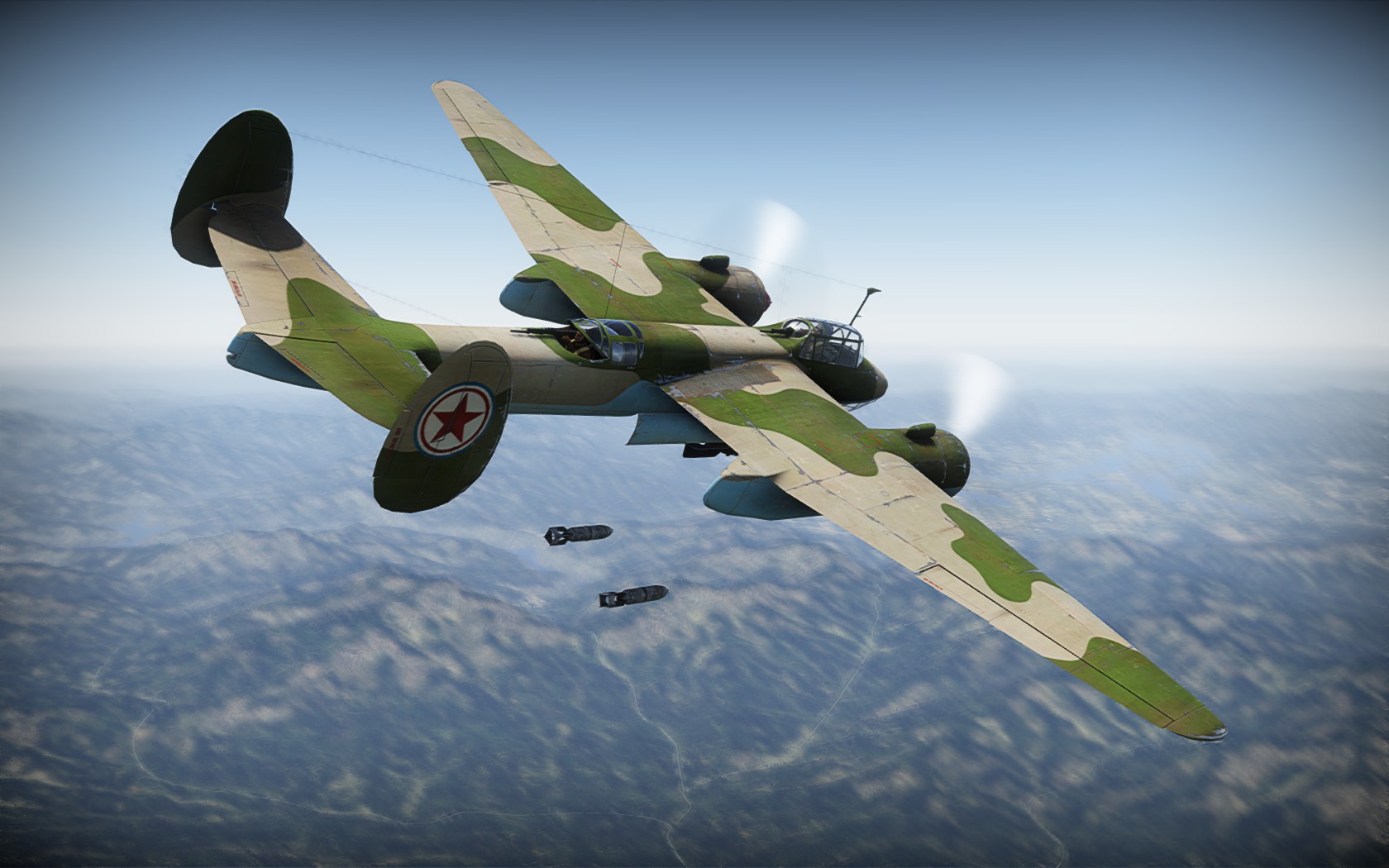This image is a highly detailed, color digital 3D rendering, likely from a video game such as War Thunder, showcasing a military aircraft in flight. The plane, which resembles a World War II era bomber, is depicted banking to the right, and is adorned with a camouflage pattern of dark olive green and light brown. The aircraft features twin propeller engines mounted on its broad wings, with the propellers visibly spinning. It also has a distinctive twin tail, and a red star set within a white circle on the right side of its tail fin. 

From the rear and right-angled perspective, visible details include the main cockpit in front and a secondary cockpit behind the wings, possibly housing a tail gunner. The plane is shown actively engaging in combat, releasing two small bombs that are visible beneath it. The scene captures the aircraft soaring over a rugged, mountainous terrain dotted with green foliage and intersected by narrow pathways, all under a mostly clear blue sky.